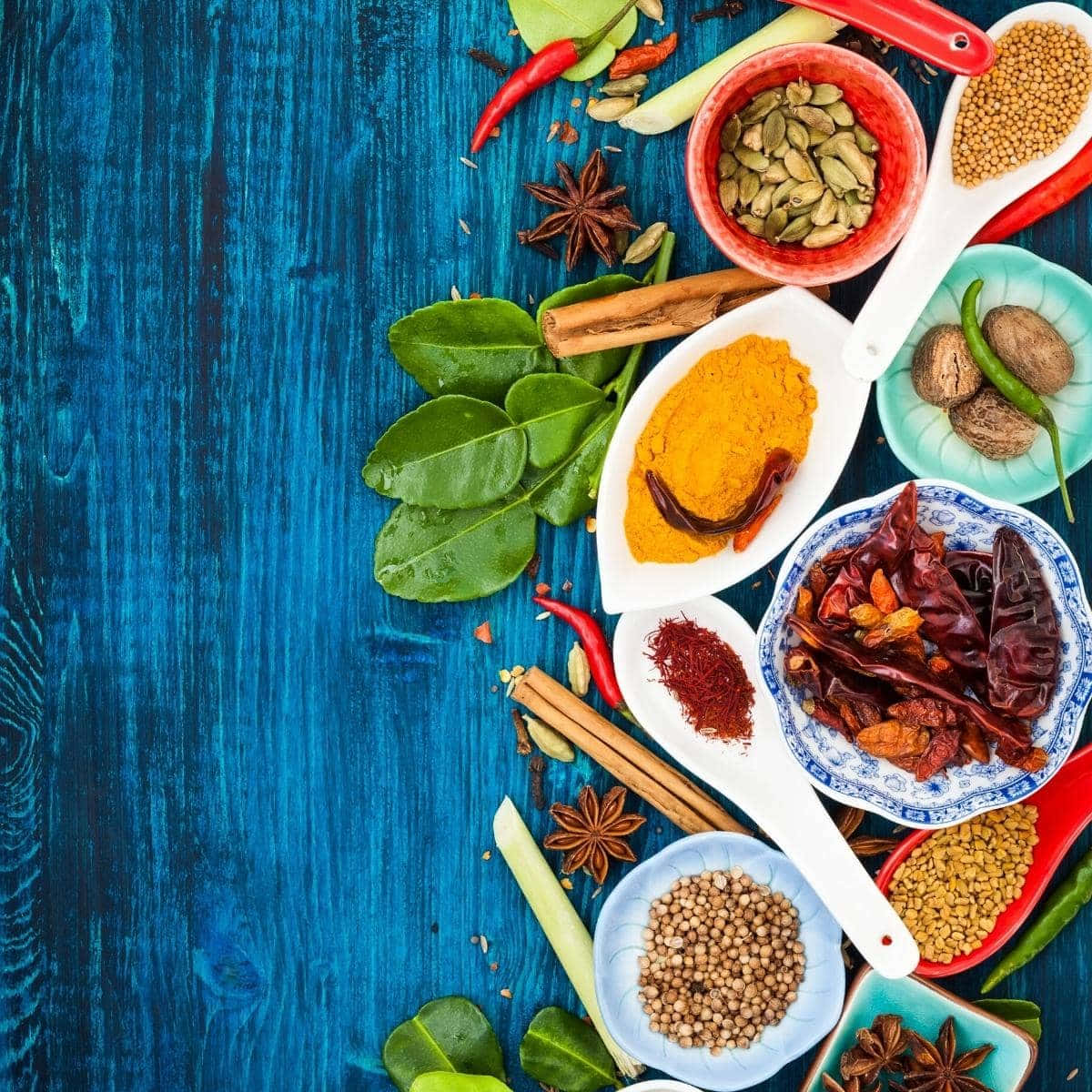In this top-down image, an array of food products is elegantly displayed on a blue wooden table. The table's blue planked surface beautifully contrasts with the vibrantly colored items atop it. On the right side of the image, from top to bottom, are several bowls and spoons containing a variety of spices, nuts, and seeds. At the top, you notice a red bowl filled with seeds beside a white spoon holding small round seeds and some red peppers. To the left of the red bowl is an anise seed pod, and just below this setup is a collection of leaves, a cinnamon stick, a white bowl with saffron in the center, and a blue bowl that houses some nuts and a green chili. Progressing towards the middle and bottom of the image, there are additional dishes and spoons, each brimming with an assortment of nuts, seeds, spices, and other ingredients, totaling around 10 different kinds. For decorative purposes, some nuts, seeds, and leaves are scattered directly on the table, enhancing the visual appeal of the arrangement.